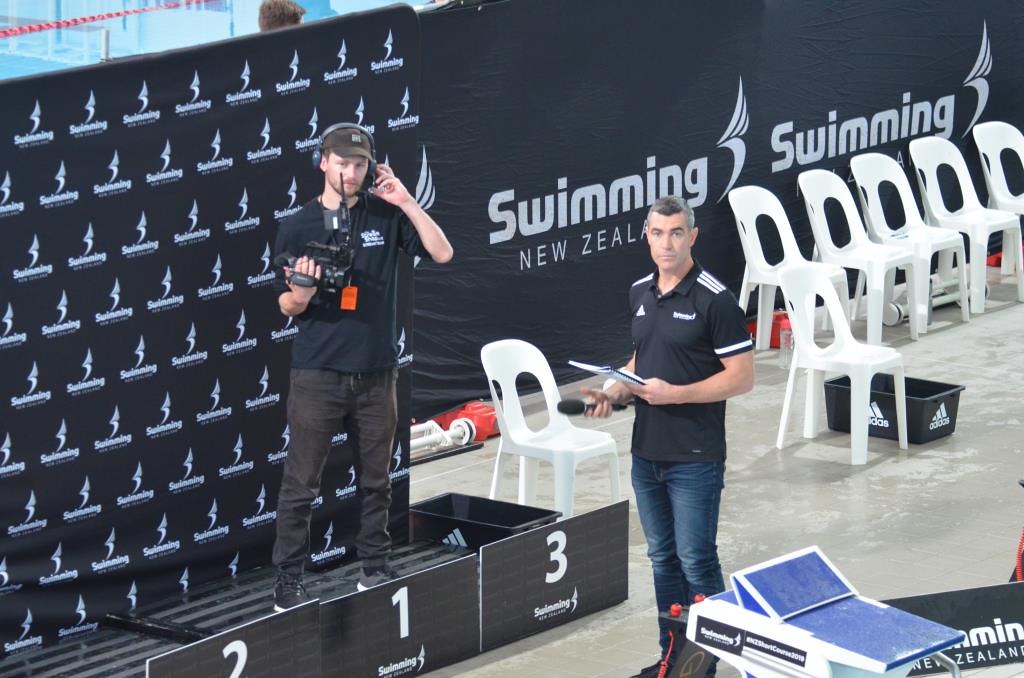In the photo, two gentlemen are prominently featured, both dressed in dark-colored polo shirts with logos. The gentleman on the left, standing atop a small podium marked with the numbers "2, 1, 3," is wearing a dark-colored baseball cap and headphones. He is equipped with camera equipment in his right hand and is adjusting his earpiece with his left. A lanyard, featuring an orange tag, hangs around his neck. His attire includes a pair of black jeans and sneakers. In contrast, the gentleman on the right wears dark blue jeans and appears to be engaged, holding a spiral-bound book in his left hand and a microphone in his right. He is looking directly into the camera. The backdrop reveals it's a swimming venue, specifically for "Swimming New Zealand," indicated by the signage. The setting includes several white plastic chairs arranged for spectators, and a black bin branded with "Adidas" positioned in front of one of the chairs. The light turquoise pool is partially visible in the top left corner, enhancing the context of a competitive swimming environment.